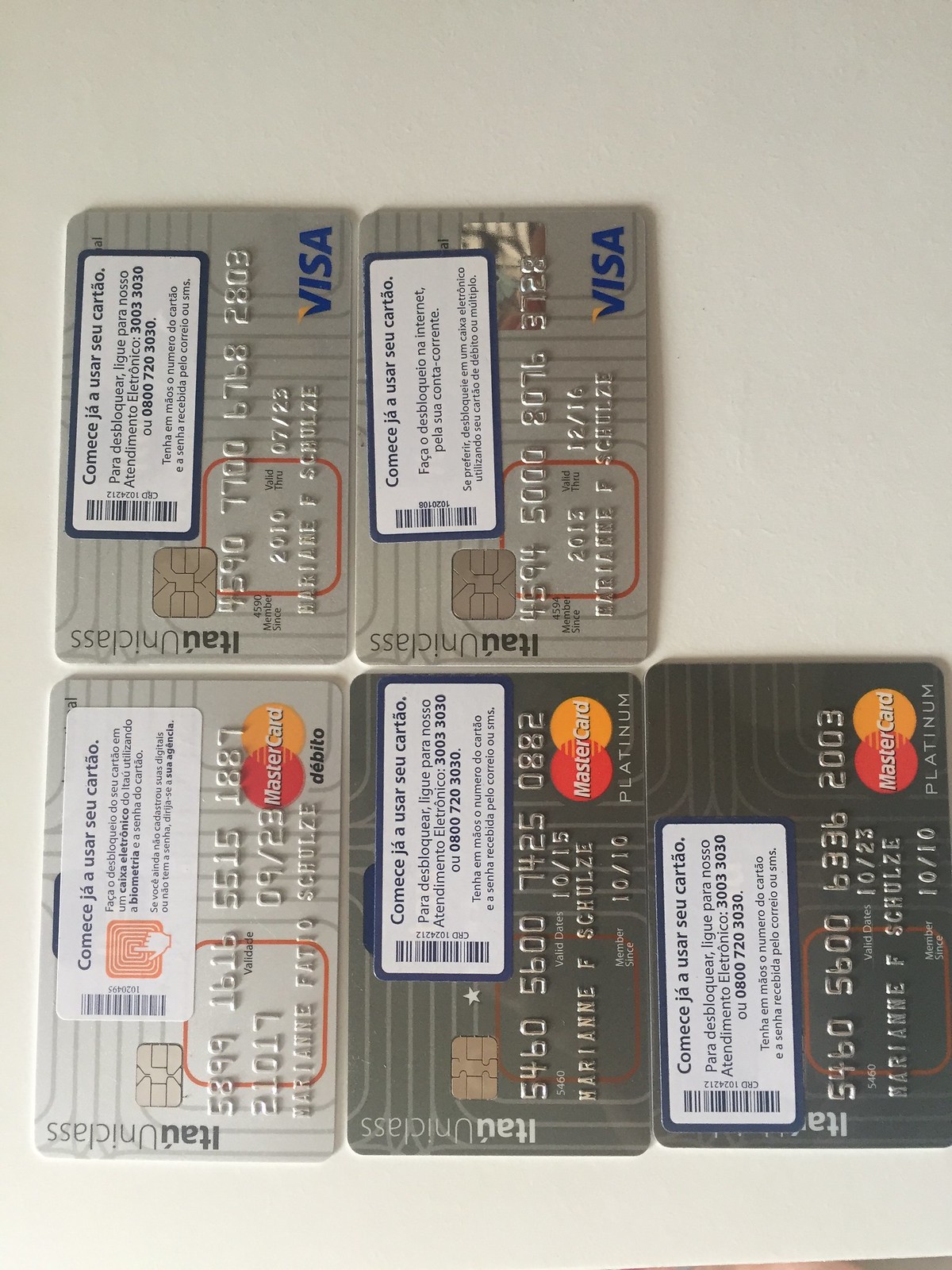This image depicts a top-down view of five credit cards arranged on a light-colored background that appears to be white, though it may have a slight gray tinge due to the lighting. The cards are aligned in two staggered rows, with three on the bottom row and two on the top row, rotated slightly counterclockwise.

Among the cards, there are two Visa cards and three MasterCards. The Visa cards, positioned on the top row, are silver with dark blue lettering. The three MasterCards occupy the bottom row. The leftmost MasterCard is silver, while the other two are platinum, distinguished by their black color and lighter text. Each card, inscribed with information in a foreign language, has the common feature of black lettering, except for the word "Platinum" which is in English on the darker cards.

Additionally, these credit cards appear to be outdated as their validity extends only until 2010 and they still bear activation stickers. The name "Marianne Schultze" appears on most, if not all, of the cards, indicating they likely belong to the same individual.